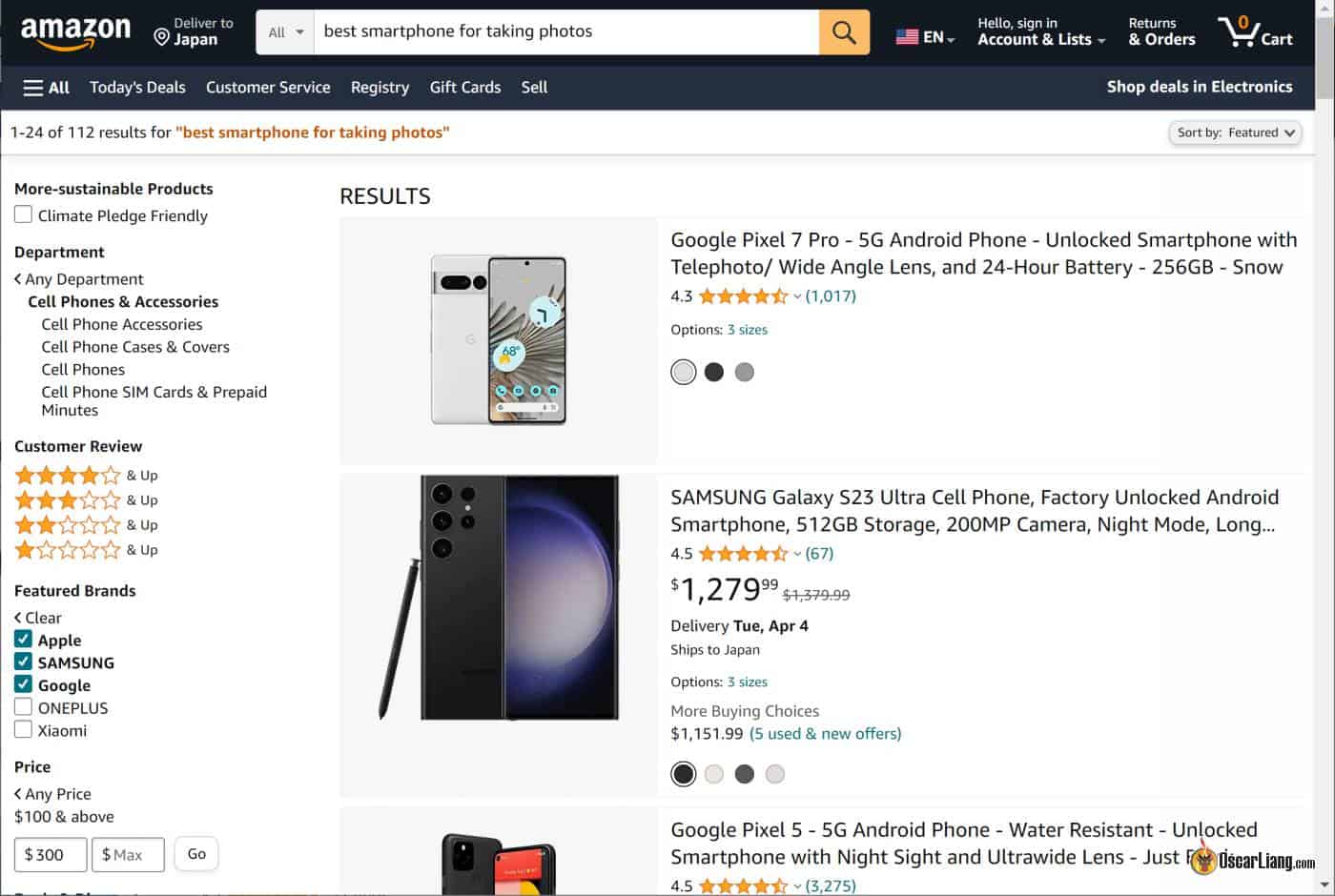This is a detailed screenshot of an Amazon.com search results page captured in a browser. The user has searched for "best smartphone for taking photos." The interface displays Amazon's signature dark navy blue, orange, and white color scheme. 

At the top, next to the Amazon logo, it indicates delivery to Japan. To the right of the logo, a search bar dominates the space, followed by language preferences set to English. Further right, standard user options such as "Hello, sign in," "Account & Lists," "Returns & Orders," and an empty cart icon are displayed. 

Below the search bar, additional navigation tabs are set within the dark blue banner, including "All," "Toys," "Today's Deals," "Customer Service," "Registry," and "Gift Cards."

The search results section indicates that 1 to 24 of 112 results for "best smartphone for taking photos" are displayed, sorted by featured products. Filters available on the left allow users to refine their search by sustainable products, department, customer review, featured brands, and price range.

Currently, three search results are visible, each accompanied by an image. The first item is the Google Pixel 7 Pro. The second result displays the Samsung Galaxy S23 Ultra cell phone, followed by the Google Pixel 5. Each listing includes details like product colors, sizes, and customer reviews.